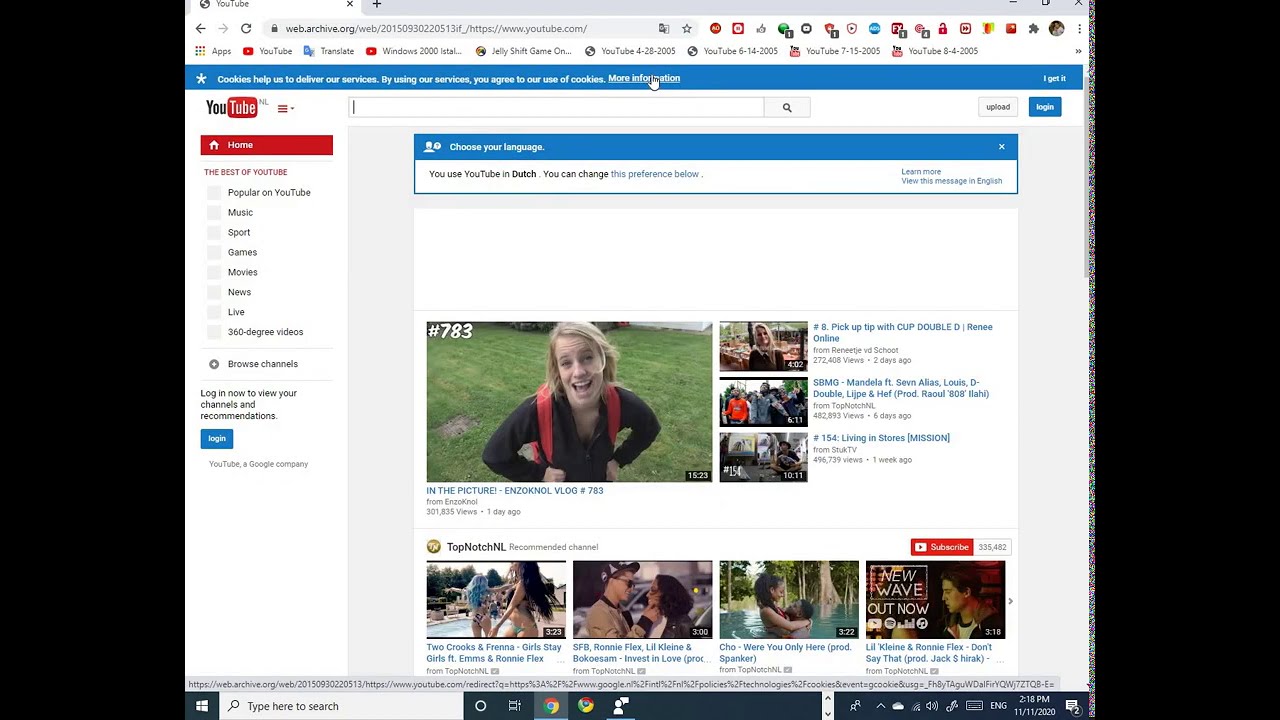This image is a wide, rectangular screenshot depicting an older version of the YouTube homepage with tall rectangular strips cropping the left and right sides. The address bar indicates the webpage is archived on webarchive.org. The top navigation bar includes standard browser icons such as the back, forward, and reload buttons, typical of an older browser interface. 

Prominently featured is a blue banner across the top of the page that reads in white font next to a star: "Cookies help us to deliver our services. By using our services, you agree to our use of cookies." This message is underlined with "more information." Below this banner, the background is predominantly white with a menu on the left side containing YouTube navigation options like "Home." The search bar is blank, and underneath, it gives an option to choose language preferences, currently set to Dutch.

In the main content area, there is a large thumbnail for a YouTube video. This thumbnail shows a blonde woman with a long-sleeve dark shirt and a red backpack standing on a green lawn, looking at the camera with her mouth open. Below this image, the text reads "in the picture - Inzoknoel vlog number 783." To the right of this main thumbnail, there are three smaller thumbnails stacked vertically for other videos. The overall webpage is filled with various colors, including white, blue, red, black, gray, yellow, brown, and assorted skin tones, providing a detailed and nostalgic glimpse into an older YouTube browsing experience.